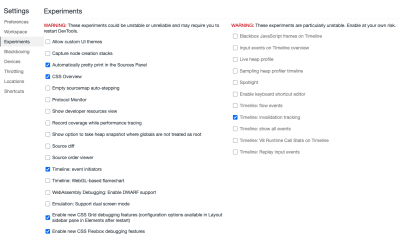The image showcases a complex user interface of a software application, seemingly related to development or debugging tools. The background of the interface is predominantly white, making the text elements stand out more. Despite the text in the background being partially obscured, specific terminologies related to experiments are discernible, such as "restarting DevTools," "allowing subject's UI," "capturing node," and "command stacks."

On the left pane of the interface, several options are visible, including "Preferences," "Workspace," "Experiments," "Locations," "Shortcuts," "Throttling," "Devices," and "Settings." A prominent red warning message adds an urgent tone to the interface. The clothing of the individual(s) in the image features white, black, and red colors, harmonizing with the interface's design elements.